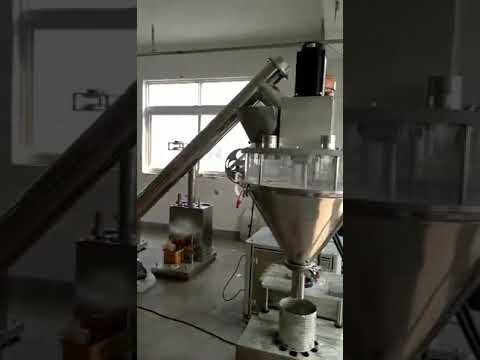The photo captures the interior of a worn and unkempt white-walled room, possibly part of a manufacturing facility or warehouse. The floors appear to be concrete, and there's piping running along the ceiling. Dominating the scene is a metallic silver funnel fixed with a nozzle, positioned on a dark gray metal or stone bench. This funnel holds a liquid that seems golden in color, although it's a bit unclear. The liquid is directed through the nozzle into a large, sturdy tin can below it. Attached to the top of the funnel is a square, block-shaped object connected to a pipe that angles down to the left. Near the top right of this assembly, there appears to be a red light partially obscured by a black cylinder. Various other pieces of mechanical equipment are scattered around the room, placed on tables. In the background, there is a large double window allowing daylight to stream in. The entire scene is intricately detailed, showing an array of industrial components and piping, with the blurred photo composition lending a sense of depth to the image.